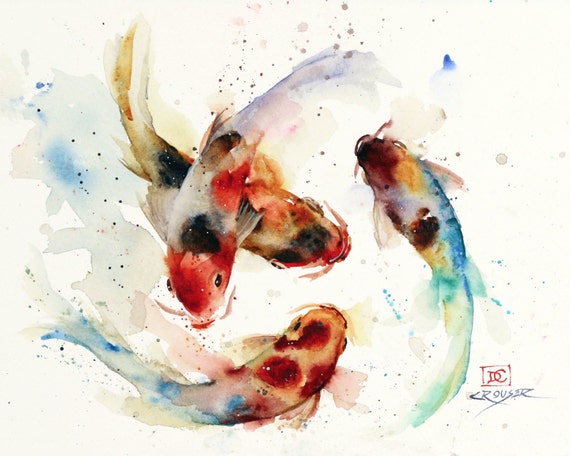This image showcases a delicate watercolor painting on a predominantly white background, depicting four intricately detailed koi fish in a circular swimming pattern. The palette features a harmonious blend of red, black, white, blue, green, and brown. Each fish exhibits unique color variations: one with blue, orange, and red hues accented by black markings along its stomach; another in the bottom left spotted with red dots; and a third with subtle brown spots, a tan body, and blue-edged fins and tail. The fish appear to float effortlessly, leaving behind trails of blue and brown bubbles. The composition is marked by a sophisticated and stylized approach, emphasizing artistic subtlety and intricate detail. The lower right-hand corner bears the signature "Krause" in blue, alongside a red symbol labeled "DC."